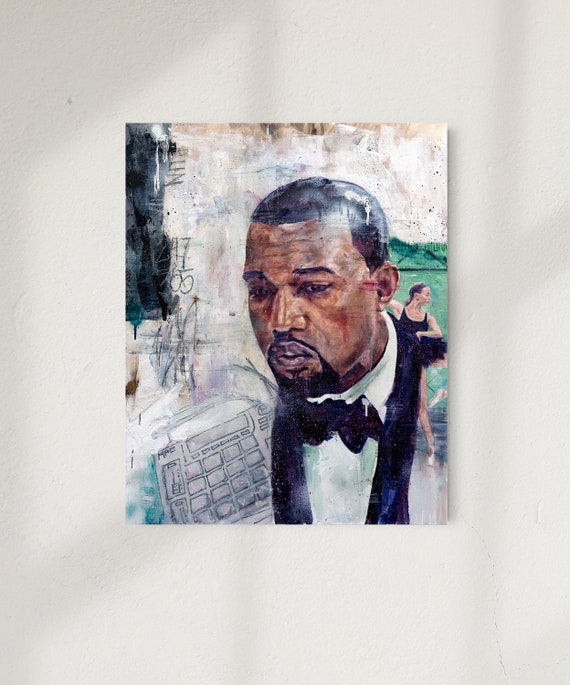The painting is a rectangular artwork depicting an African-American man, reminiscent of Kanye West, with short black hair, a mustache, and a goatee, trimmed very thin. He wears a black tuxedo with a white shirt and a black bow tie, his expression somber. To the lower left of the man’s face, there is a depiction of an object resembling a game controller or calculator, featuring multiple buttons and a screen on top of it.

To the right of the man, near his ear, stands a white female ballet dancer with brown hair. She is dressed in a black outfit with a black tutu and white ballet shoes, one long leg elegantly extended out. The background behind her is light green, suggestive of a green door. The overall background of the painting is predominantly off-white with black patches, creating a splotchy effect.